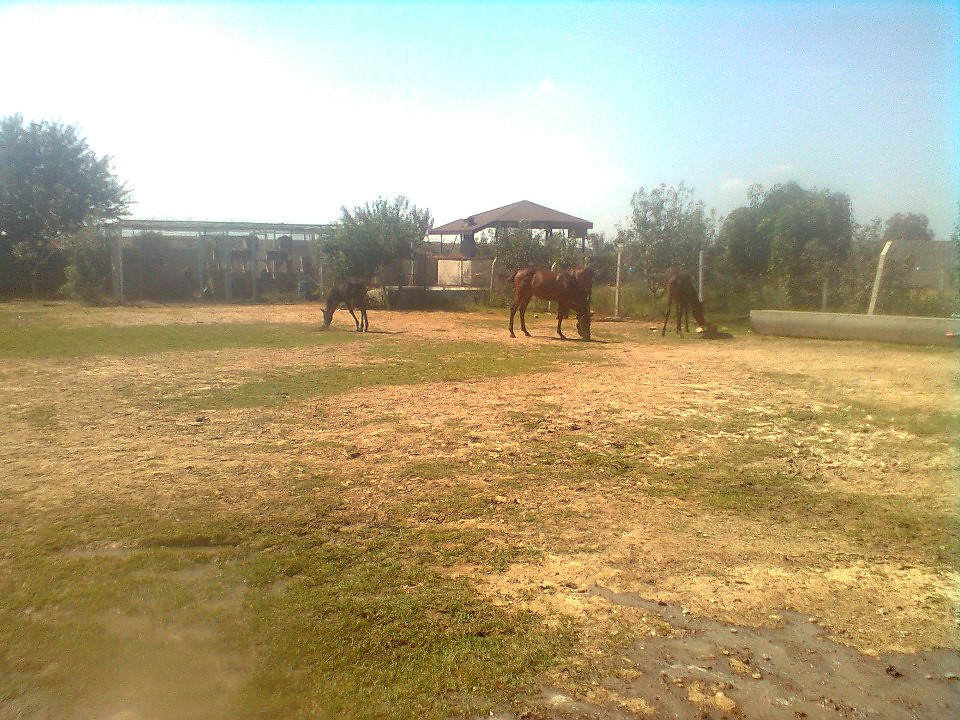In this bright, sunlit photograph taken on a farm, the foreground features a mixture of sparse, partly green, partly dead grass interspersed with rocks and dirt, as well as muddy puddles. Four horses are seen grazing in this field: three chestnut brown horses with black manes and close-cut tails in the mid-center, and a smaller, younger, almost black horse to their left. Each horse has its head down, immersed in grazing, except for one brown horse with a white head standing watchfully in the background. Behind the fence in the background, there's a small building with a triangular-shaped, dark brown roof and an indistinct open structure, possibly serving as horse stalls or storage. To the left and right of the structures stand large trees and bushes, under a partly cloudy light blue sky with fluffy white clouds. A horizontal metal object, likely a water trough, is also visible to the right of the grazing horses.